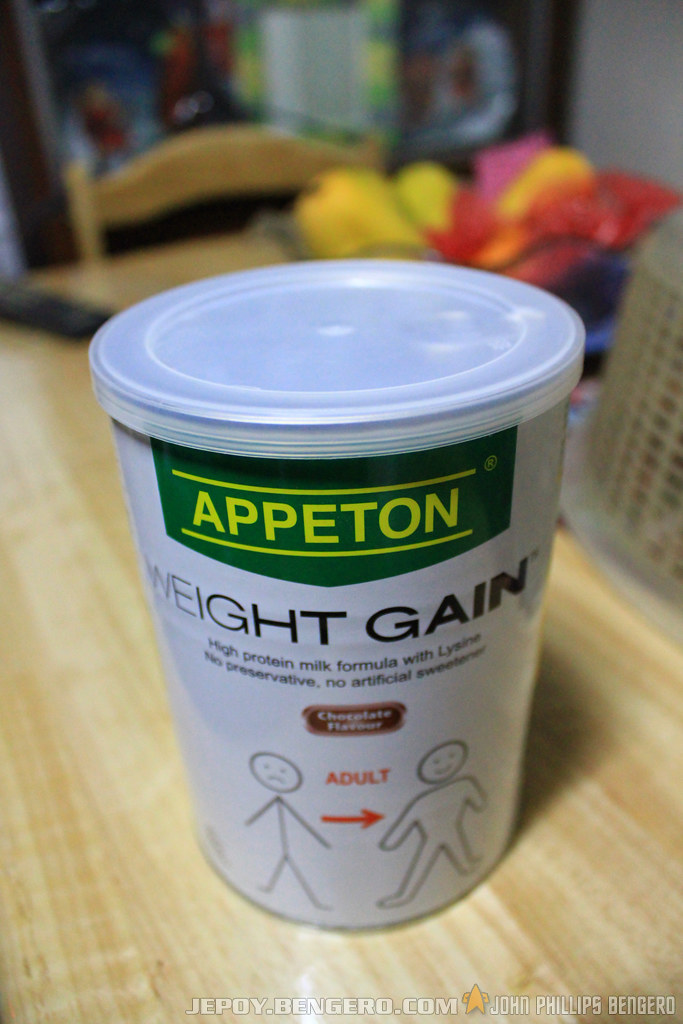The image showcases a can of Appeton (spelled A-P-P-E-T-O-N) Weight Gain, prominently labeled as a high-protein milk formula with lysine. The product boasts no preservatives and no artificial sweeteners and is available in a chocolate flavor. The can features an emblem depicting a transition from a frowning stick figure labeled "ADULT" in red capital letters—with an arrow pointing to the right—to a fuller-bodied, smiling figure.

The can is placed on a wooden dining or kitchen table. In the background, there is an upside-down laundry basket and possibly some clothes, though they are blurred and out of focus. At the bottom of the image, the text "JEPOY.BENGERO.com, John Phillips Bengiro," is visible.